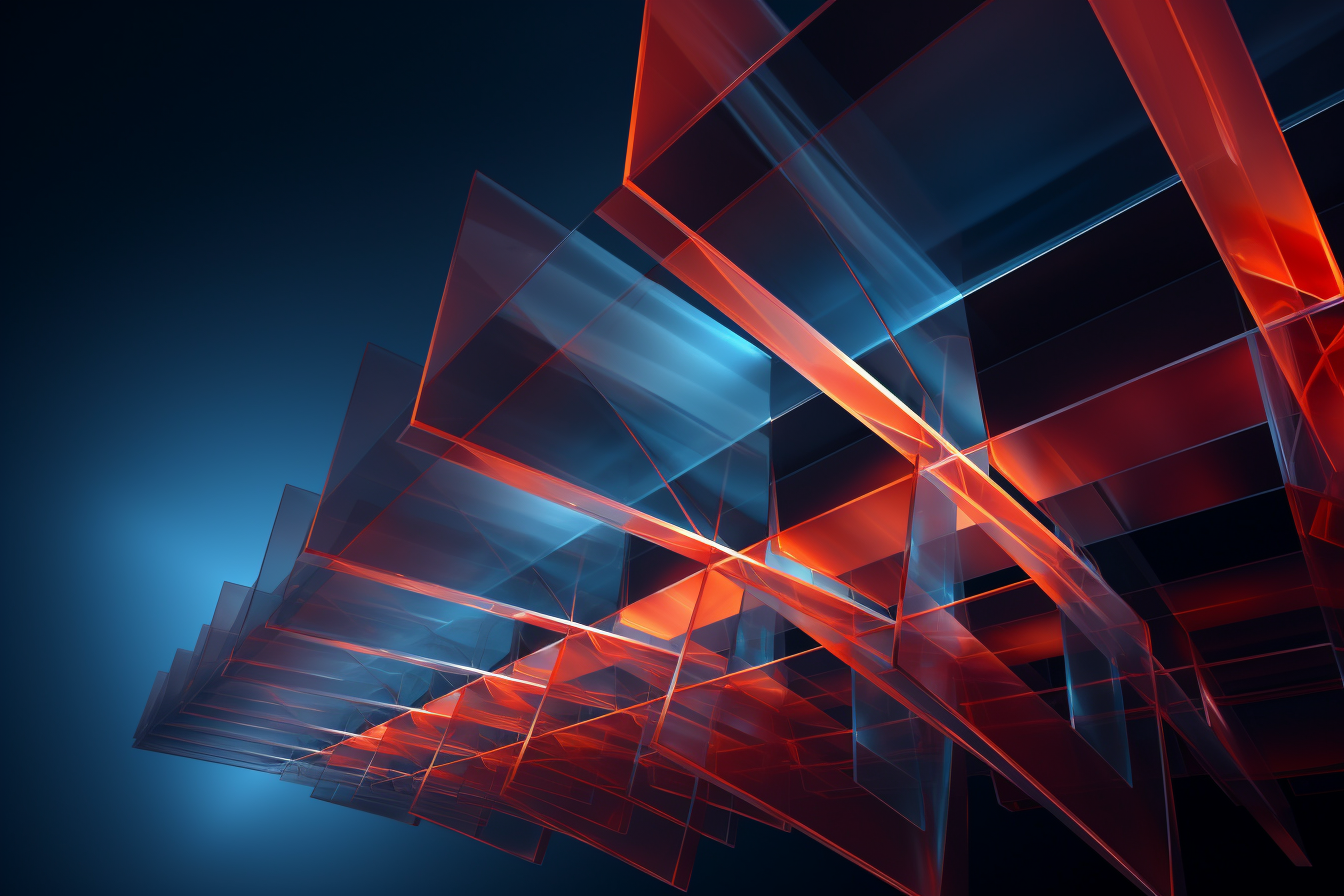The image appears to be an abstract digital rendering with a dark blue background. Dominating the composition are box-like shapes that align in three distinct rows, positioned off-center towards the right. These shapes have glowing red outlines and exhibit a striking interplay of colors including dark blue, light blue, red, and orange. Adding to the abstract quality, the shapes resemble a glass shelf or ledge emerging from the lower right corner. The translucent, glass-like appearance of these shapes allows for a blue sheen to be visible over the predominant orange color. No context or scale is provided, leaving the true nature and dimensions of the object open to interpretation. The overall design is purely abstract, with no textual elements present.